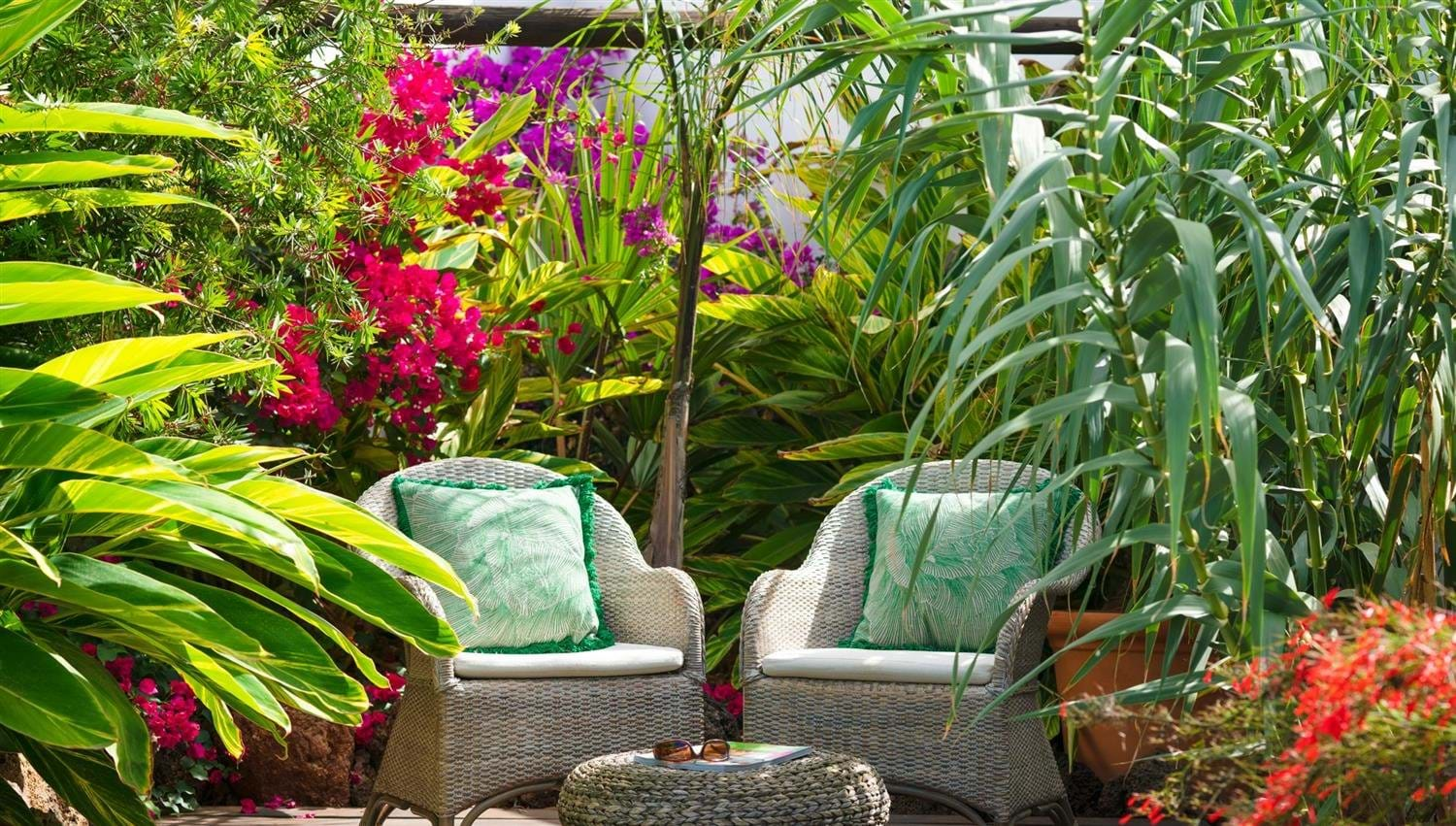In this detailed landscape-oriented color photograph, two white wicker chairs with green floral pillows and tassels are positioned in a picturesque garden setting. Facing each other towards the middle of the image, the chairs flank a round white wicker ottoman table, partially visible at the bottom. The table holds a pair of bronze-lensed sunglasses with black rims and a book. The scene is lush, framed by a white fence in the background with a bluish-white sky above. Surrounding the chairs are a variety of plants and flowers: tall fronds reminiscent of corn stalks, red and purple flowering shrubs, and large banana leaves. Notably, red flowers trail from a terracotta planter to the right of the right-hand chair. The ground appears rocky, adding to the rustic charm of this garden retreat. This photographic representation captures the tranquility and vibrant plant life of an inviting outdoor setting.